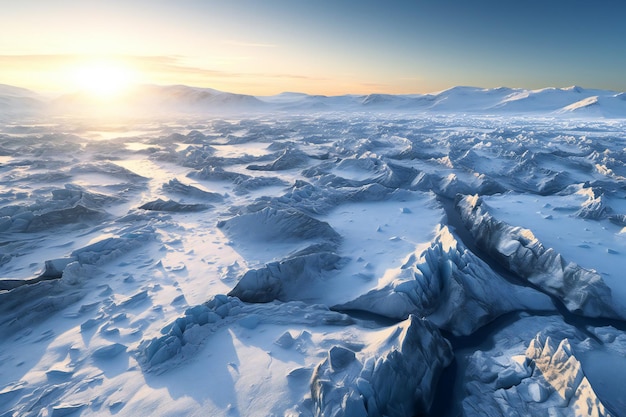This digitally rendered image, captured from a high vantage point, depicts a vast, snowy, and icy landscape bathed in the hues of sunrise. The scene is dominated by flat, snow-covered plains interspersed with rocky cliff textures. In the distance, a ridge of snow-covered mountains lines the horizon, with the sun just beginning to rise over the left side of the frame, casting a soft yellow glow and illuminating the sky with subtle pink clouds. The ground below is a mosaic of glacial chunks and sharp ridges, with sections of bright white snow giving way to bluish shadows. Crevices between the icy formations hint at flowing water or melted ice, adding to the textured and somewhat surreal appearance of the landscape.